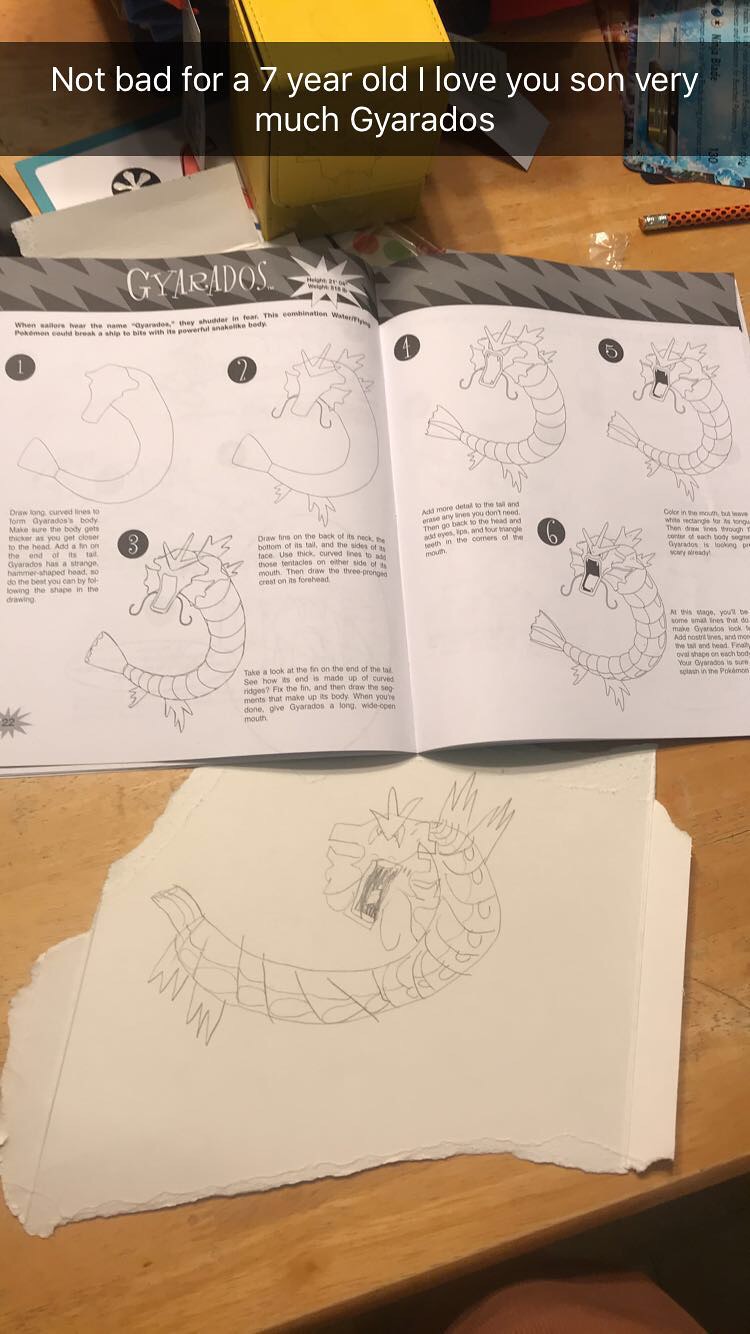The photograph captures a well-lit, indoor scene focused on a wooden table. At the center, a white instructional book is flipped open, detailing six steps to draw a unique dragon-fish hybrid creature. This creature has a dragon head and a fish-like flipper at the tail. Each step is illustrated with increasing detail and accompanied by paragraphs of guidance. Above the book is a black banner with white text that reads, "Not bad for a seven-year-old. I love you, son, very much. Gallardos."

Below the book, a torn piece from the back of a box serves as a makeshift drawing surface. On this white cardboard, someone has sketched the dragon-fish creature in pencil, closely following the book's instructions. The drawing is noticeably well-executed considering it's done by a seven-year-old. Scattered on the table are a pencil tip and a yellow box, adding to the scene's authenticity and homely feel. The overall composition is sharp and clear, emphasizing the effort and affection conveyed in the creation of the drawing.